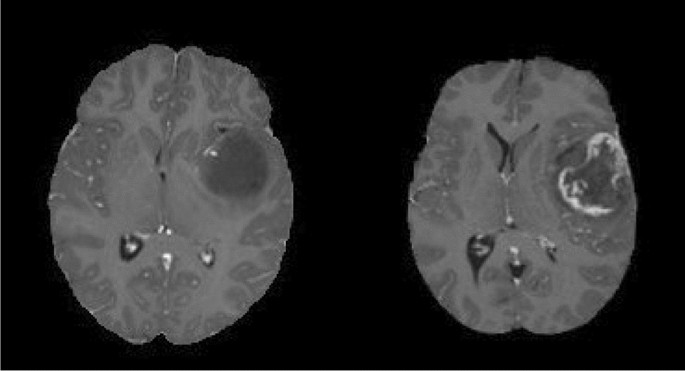The image presents two detailed grayscale brain scans viewed from the top, both set against a solid jet black background. The scan on the left features distinct gray and dark gray modeling that outlines the brain's structures, with a notable circular gray object in the upper right quadrant. Further detailing includes a white-centered dark circle in the lower central area of the left hemisphere, a prominent white line running through the center, and a small white dot located in the right hemisphere. On the right scan, the corresponding major area, originally depicted as a large gray dot in the left scan, now appears as a flat white region. Additionally, the lower area that once had a dark circle with a white center on the left brain is now heart-shaped with a dark center. The central white line has evolved to be broader and displays an additional dark area above it, while the white mark on the far right remains although it has changed shape. The fine ridges of the brain are visible through gray lines in both scans, and the overall image shows the hemispheres clearly, despite a few white specks throughout. No text accompanies the image.